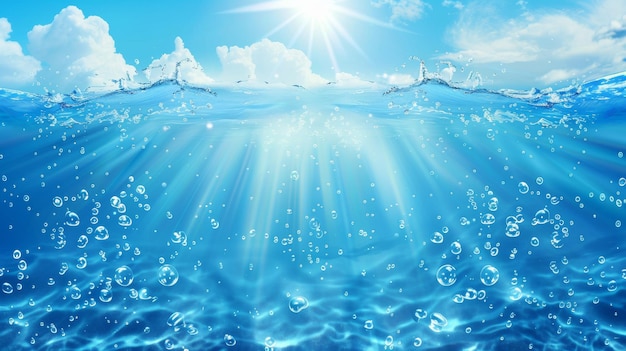This vibrant and beautiful image captures a breathtaking scene of the ocean under a clear, blue sky with scattered white clouds. At the heart of the composition, the brilliant sun shines brightly, its radiant rays piercing through both sky and water. One-third down from the top, the serene blue sky gives way to the ocean, where a large wave surges powerfully, sending splashes and bubbles into the air. The crystal-clear water reveals intricate details: luminous sun reflections shimmering on the surface, smaller ripples beneath the primary wave, and scattered air bubbles that add texture and life. The overall clarity of the water even hints at the ocean floor below, making the entire scene feel pure and untainted.